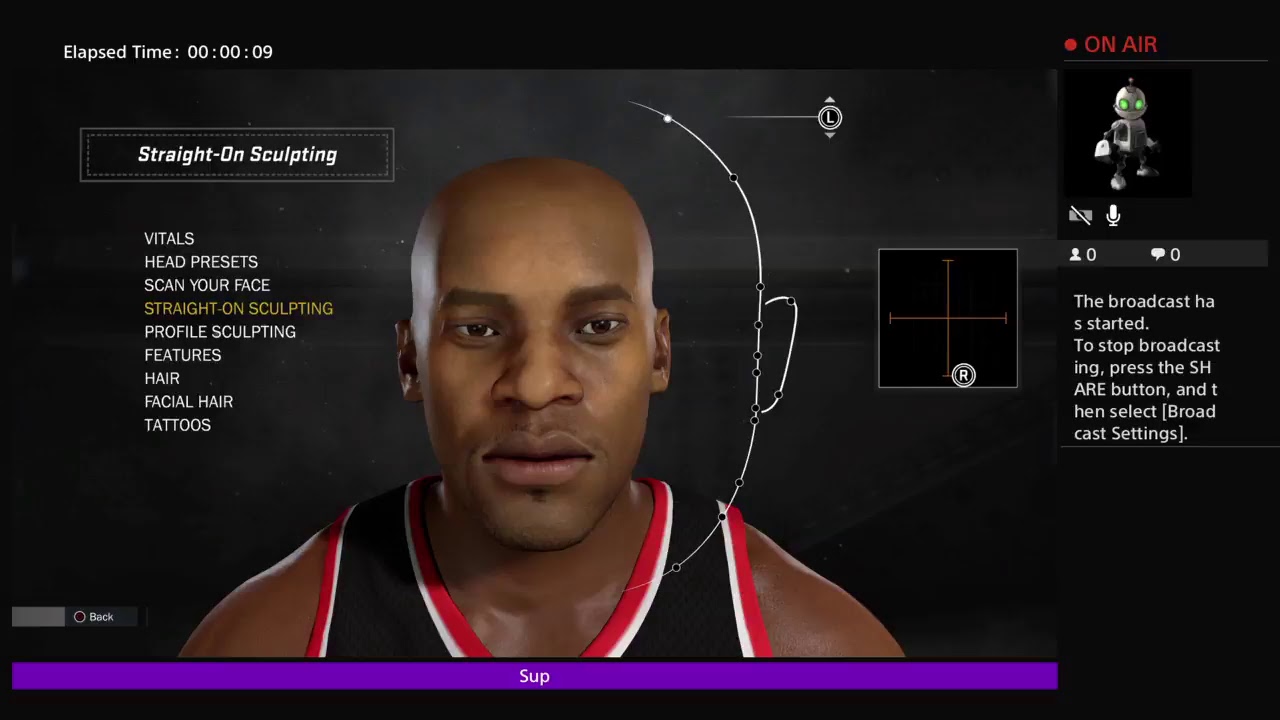The image appears to be a screenshot from a character designing interface, likely from a video game. At the top left corner, the text "Elapsed Time: 00:00:09" is displayed, indicating the session duration. On the top right, the word "On Air" is highlighted in red, suggesting the session might be live-streamed or recorded. In the center of the screen, a bald character wearing a black jersey with white and red outlines is prominently shown. On the left side of the interface, there is a menu with various options- "Vitals," "Head Presets," "Scan Your Face," "Straight On Sculpting," "Profile Sculpting," "Features," "Hair," "Facial Hair," and "Tattoos," with "Straight On Sculpting" currently selected.